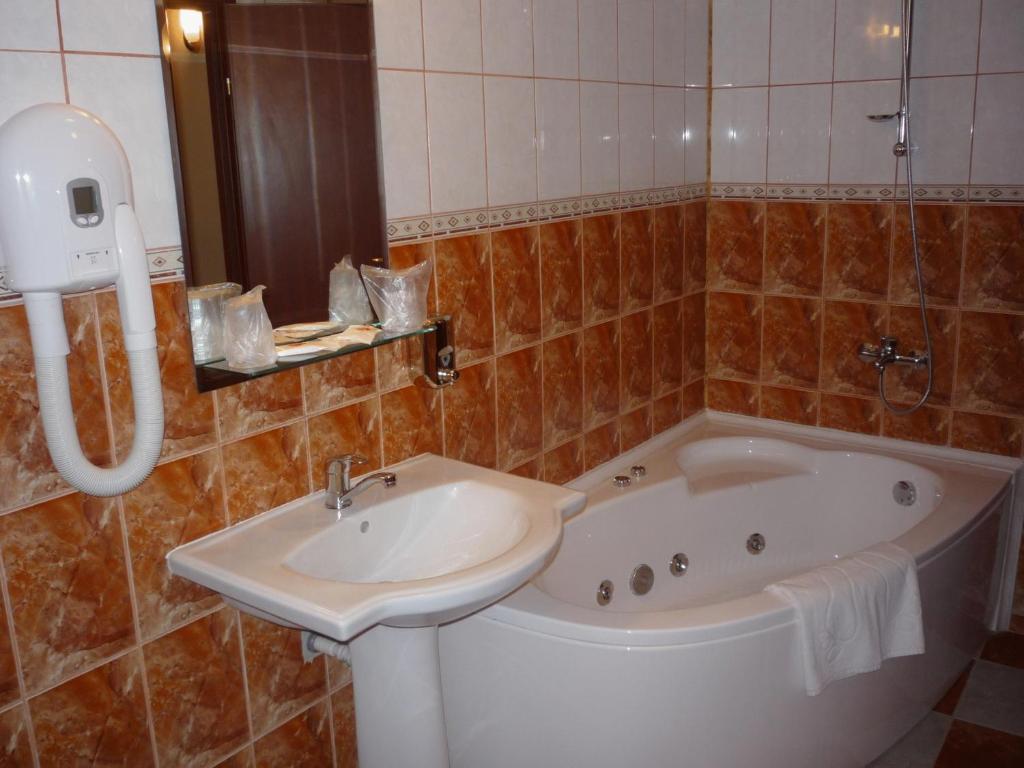This is a detailed horizontal photograph of a bathroom, likely from a hotel, indicated by its amenities and arrangement. The room features a freestanding white sink with a mirror positioned above it. The mirror includes a shelf holding two cups sealed in plastic. To the left of the sink hangs a dated hair dryer. The plumbing of a shower head extends upwards from the bathtub area, though the head itself is not visible. The bathtub is a white, jetted model with an ovular internal shape, and a towel draped over its edge. The walls are adorned with a combination of brown marbled tile on the lower half and plain white tile on the upper half, separated by a decorative border. The floor consists of a checkered pattern of white and brown tiles. The mirror's reflection reveals a light bulb and additional wall details, contributing to the room's illuminated, cozy ambiance. The unique combination of fixtures and decor elements, such as the dual-tone tiles and dated apparatus, provide a vintage yet functional appeal.